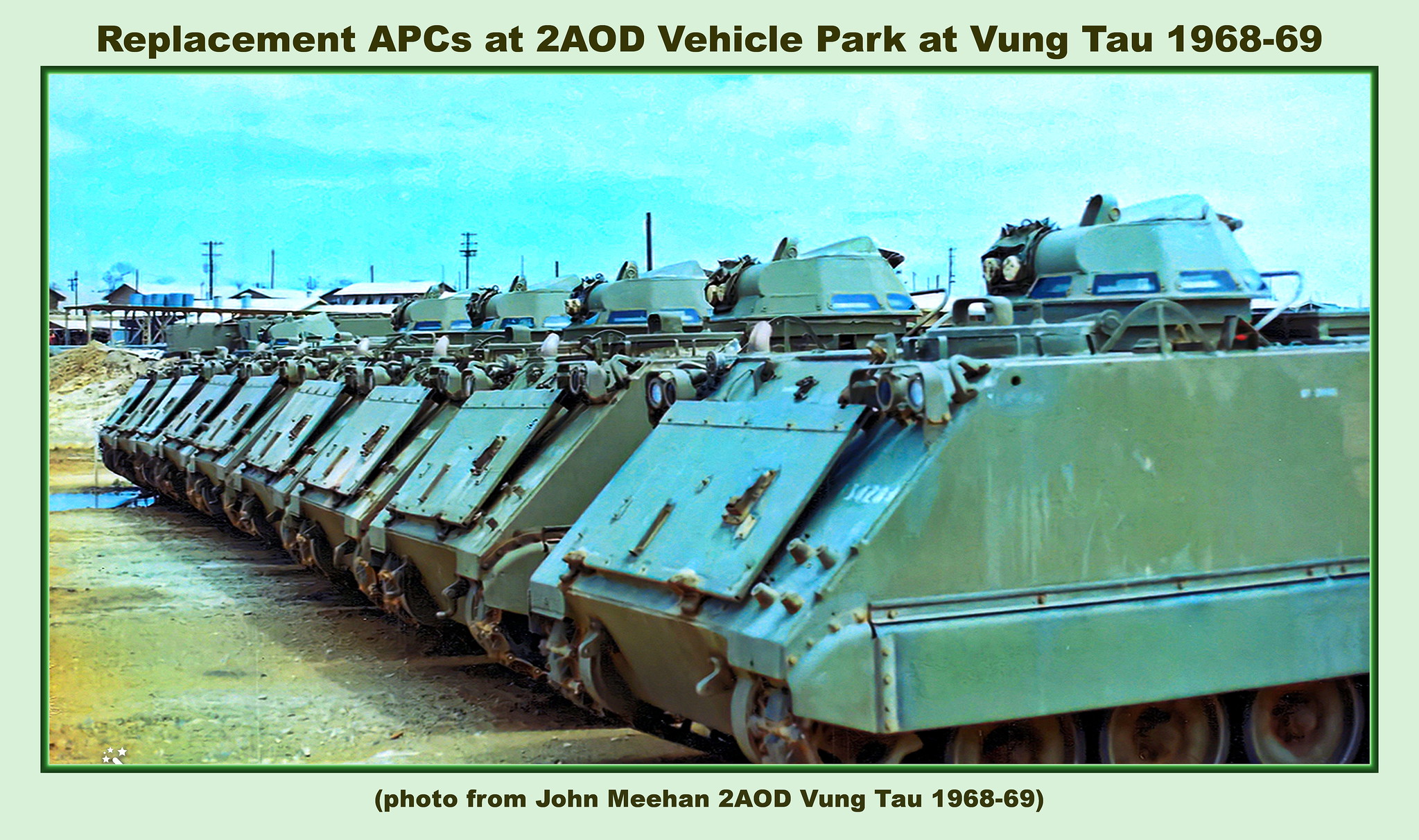The photograph, framed by a light green border with a darker green inner frame, prominently features a lineup of nine tanks, retrofitted to look like vintage military vehicles from the late 1960s. Captioned at the top and bottom, the text reads: "Replacement APCs at 2AOD Vehicle Park at Vung Tau, 1968-69. Photo from John Meehan, 2AOD Vung Tau, 1968-69." The tanks, bearing signs of wear and weather exposure, are arranged in a neat row, traversing a muddy field with noticeable puddles. The backdrop reveals an army base, suggesting the location to be Vung Tau, Vietnam, captured in broad daylight, with the colors green, yellow, brown, tan, light blue, white, and gray vividly marked throughout the image.